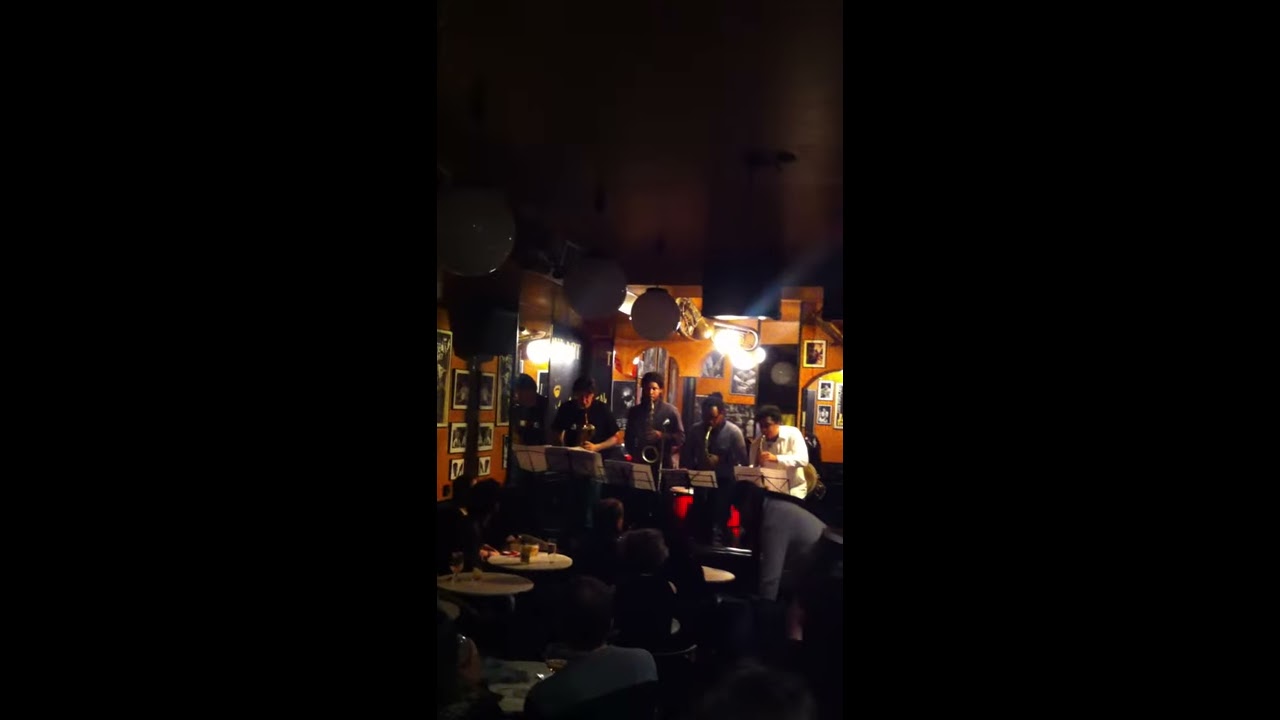In a dimly-lit indoor setting that resembles a bar or a restaurant, numerous round white tables are scattered across the room, each occupied by patrons. Drinks adorn the tables, although food is scarcely seen. The venue, bathed in a shadowy ambiance, features large globe lights hanging from the black, shiny ceiling, all switched off. The walls are painted orange and adorned with black and white photographs, adding to the artistic vibe of the space. 

A band of five musicians stands at the forefront, all donning black and white attire. Each musician is positioned behind a music stand, and they are engaged in playing what appear to be saxophones and clarinets. The rightmost musician stands out in a white top, while the others sport darker outfits. Interestingly, one musician on the far left seems to be in motion, possibly entering the scene late or not being part of the group.

The audience's attention is firmly fixed on the band, creating an intimate atmosphere heightened by the closeness of the tables to the performers. One woman, likely a waitress, leans over a table on the right side of the room, adding to the bustling, yet cozy environment. The backdrop behind the musicians includes a wooden wall punctuated by a possible mirror that reflects some light not captured in the image, hinting at an off-camera light source. The entire scene is captured in a color photograph with wide black bands on the left and right, suggesting it was taken in portrait mode on a cell phone.